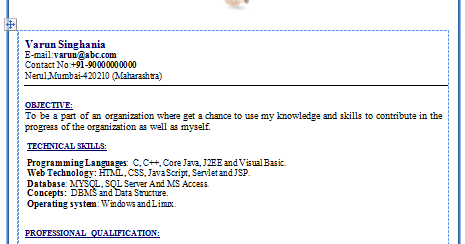In this image, an email message draft is displayed against a simple white background. The sender's name, "Varun Singhania," and email address, "varun@abc.com," are clearly visible. Below this, the contact number "+91-9000000000" is listed. Further down, the locale information reads "New World, Mumbai-420210, Maharashtra."

At the top of the content section, it appears to be part of a resume. The "Objective" statement reads: "To be a part of an organization where I get a chance to use my knowledge and skills to contribute to the progress of the organization as well as myself."

The image also lists "Technical Skills," including:
- **Programming Languages:** C, C++, Core Java, J2EE, and Visual Basic
- **Web Technologies:** HTML, CSS, JavaScript, Servlet, and JSP
- **Databases:** MySQL, SQL Server, and MS Access
- **Concepts:** DBMS and Data Structure
- **Operating Systems:** Windows and Linux

At the bottom of the page, a heading titled "Professional Qualifications" is visible, although specific details under this section are not shown in the image.